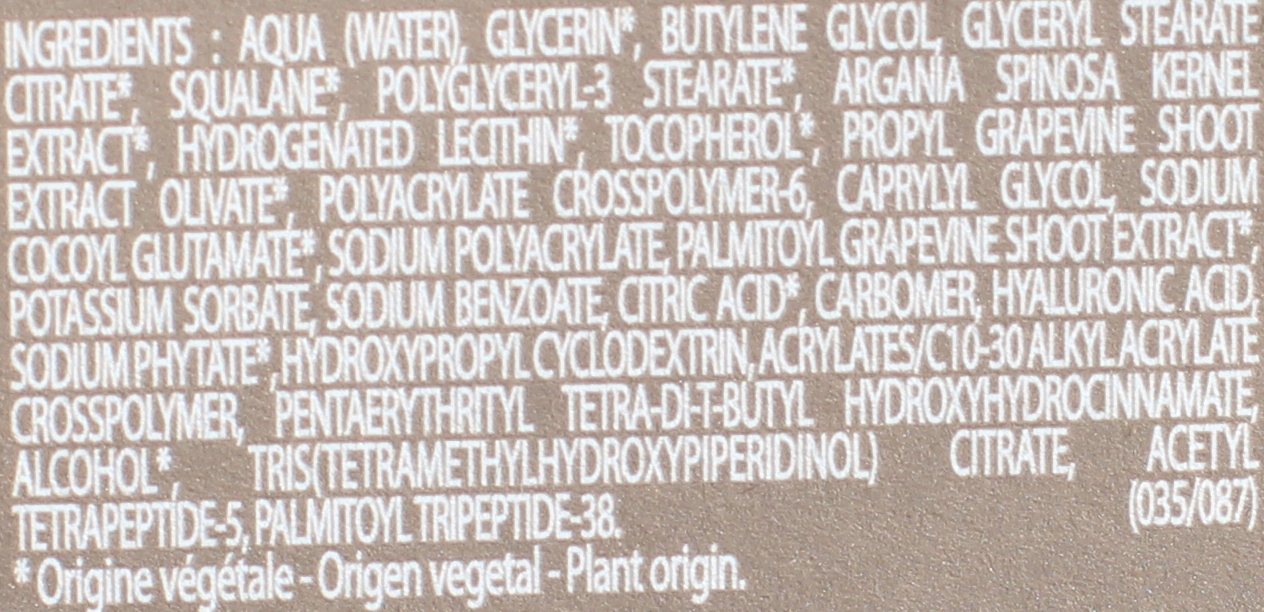The image displays a highly detailed, zoomed-in view of a nutrition label focused specifically on the ingredients list. The label is set against a tan background with white lettering, making the text clear and legible. The list of ingredients includes: Water, glycerin, butylene glycol, glyceryl stearate citrate, squalene, polyglyceryl-3 stearate, argania spinoza kernel extract, hydrogenated lecithin, tocopherol, propolis, grapevine shoot extract, olivate, polyacrylate crosspolymer-6, caprylyl glycol, sodium potassium sorbate, sodium benzoate, citric acid, carbomer, hyaluronic acid, sodium phytate, hydroxypropyldextrin, aceroloyl cerate-C10-30 alkyl acrylate crosspolymer, pentaerythrityl tetra-di-t-butyl hydroxyhydrocinnamate, alcohol, tris (tetramethylhydroxypiperidinol) citrate, acetyl tetrapeptide-5, and palmitoyl tripeptide-38. 

On the right side of the label, enclosed in parentheses, is the code "035-087" followed by an asterisk symbol (*). Below this code, the phrase "Origin: Vegetable. Plant Origin." is printed, indicating that the ingredients are derived from plant sources.